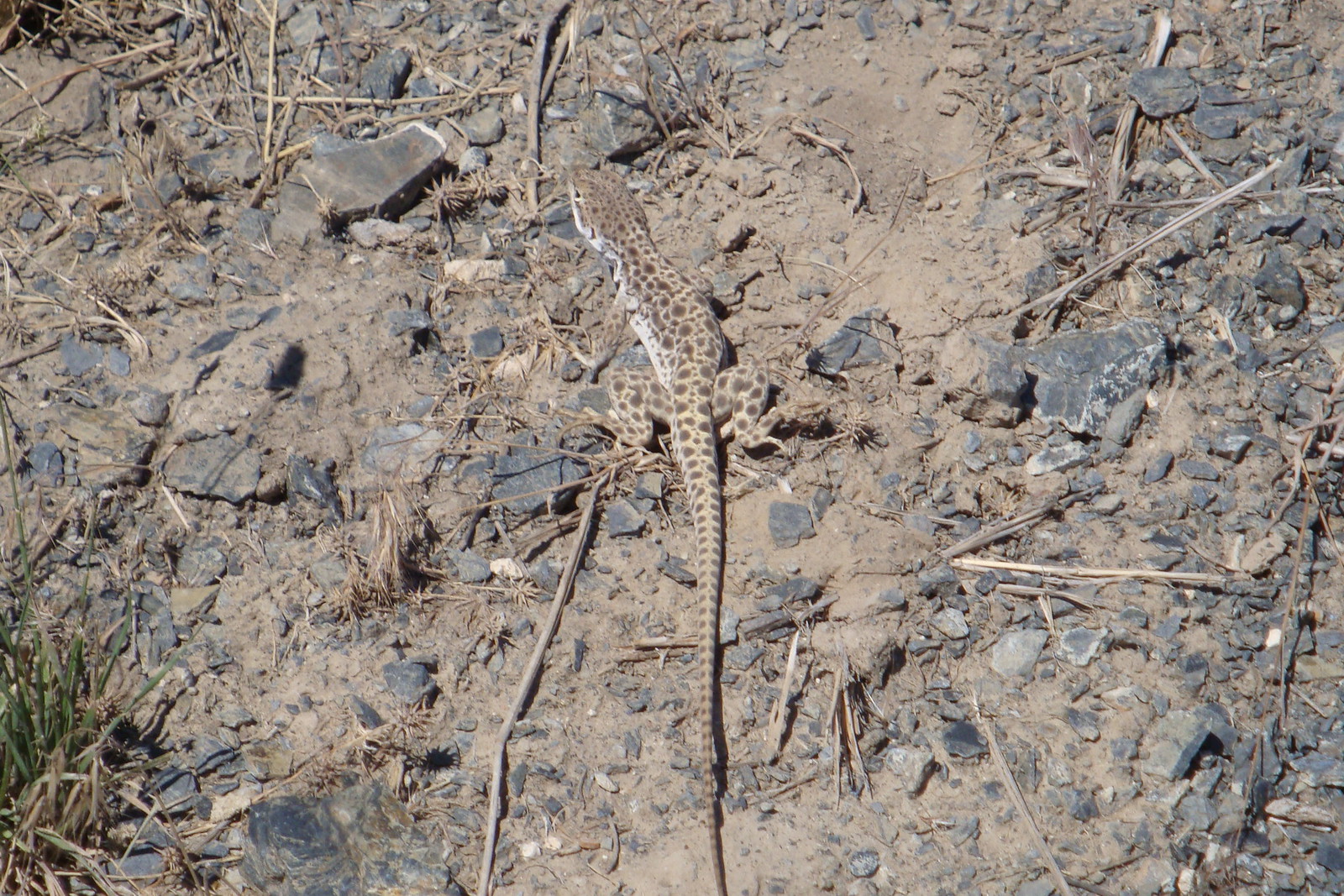This image, taken outdoors, presents a top-down view of a small, camouflaged lizard, possibly a gecko, blending seamlessly into its arid surroundings. The ground is mostly barren, composed of a sandy, pale brown terrain with scattered patches of dead grass and occasional green grass to the side. Among the slate-colored rocks and sparse, dry shrubbery are some darker rocks resembling charcoal. The lizard, whose body features a mottled pattern matching the ground's color, has a long tail and is positioned facing away from the camera, demonstrating effective natural camouflage in this scrubby, desolate environment.